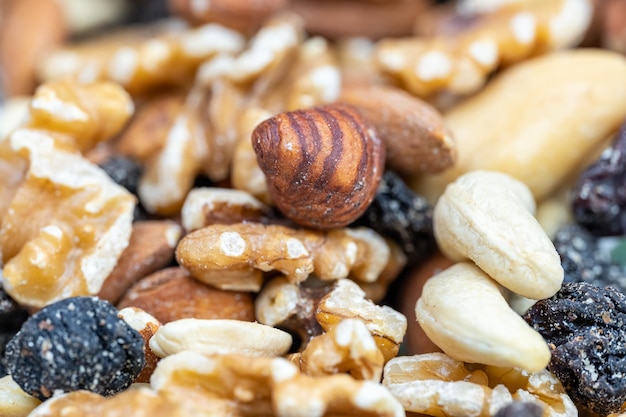This highly detailed close-up photograph showcases an assortment of mixed nuts and raisins. In the foreground, each nut and raisin is in perfect focus, capturing intricate textures and details. The background, though slightly blurry, still reveals more nuts, maintaining the theme throughout the image. Specifically, the scene includes an intriguing Brazil nut, which has peculiar lines giving it an unusual appearance resembling a caterpillar cocoon. Surrounding it are pieces of cracked walnuts, and a couple of cashews stacked together are positioned to the lower right. Small, brain-like raisins are scattered, some covered in fine peanut particles or "nut dust." The nuts exhibit a range of brown and cream colors, suggesting a crunchy, edible assortment. Despite some initial confusion with stones and shells due to the photorealistic quality, the image clearly represents a variety of mixed nuts and raisins, perfectly assembled and visually striking.